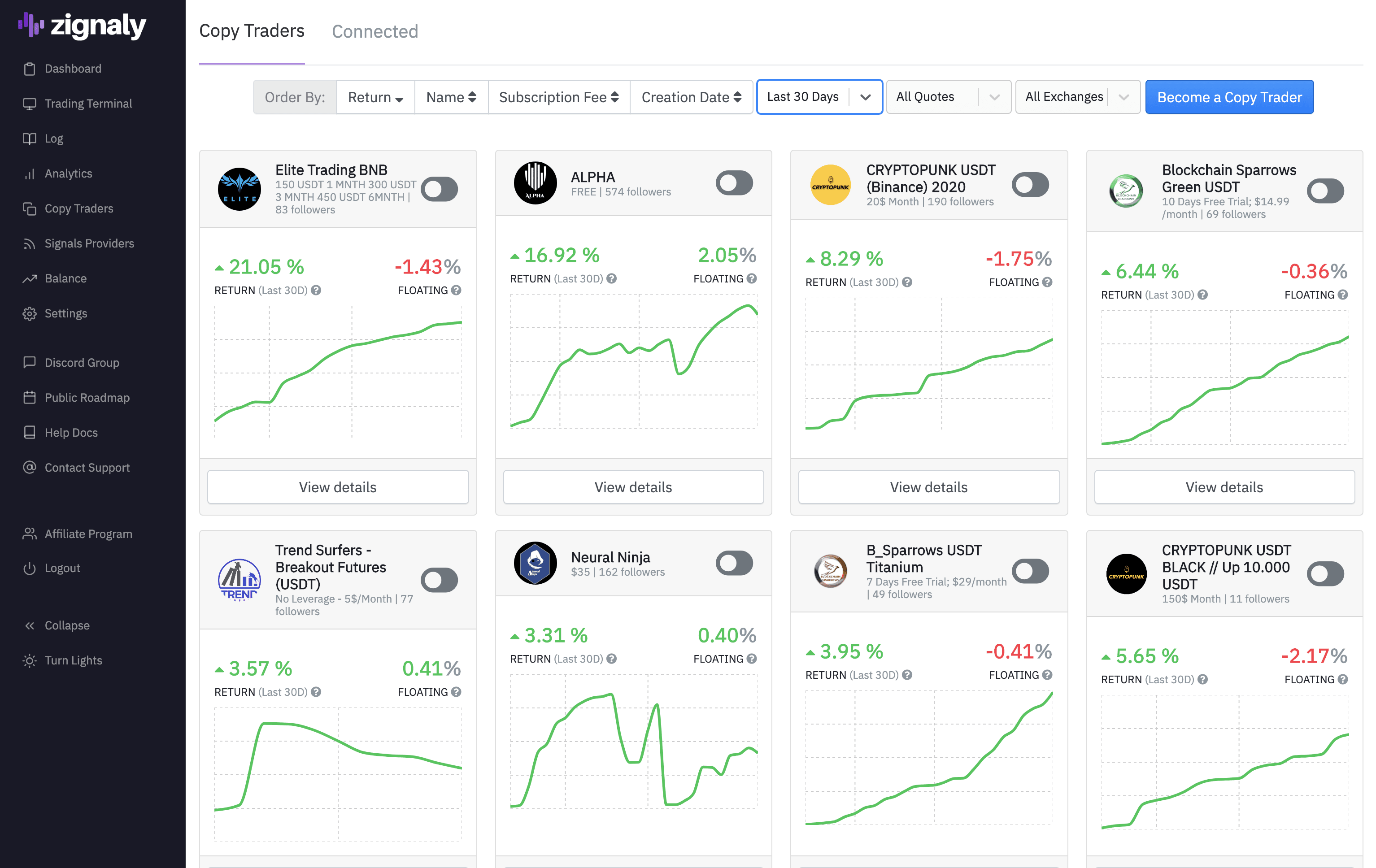This image captures a screenshot from the Zignaly platform, which can be accessed via either its website or app. In the top-left corner, there is a distinctive purple logo resembling a sideways 'Z', accompanied by the word "Zignaly" written in white on a black background.

The left side of the interface features a sizable black vertical column containing an extensive menu of categories. These categories, listed beneath the Zignaly logo, include Dashboard, Trending, Trading Terminal, Log, Analytics, Copy Traders, Signal Providers, Balance, Settings, Discord Group, Public, Roadmap, Helpdesk, Contact Support, Affiliate Program, Logout, and Collapse. Each category is paired with its own icon, and there are options to adjust the column's size and toggle between light and dark modes.

The main section of the image, situated to the right and occupying the majority of the space, is set against a white background. The top part of this section displays the "Copy Traders" tab, which is highlighted in blue to indicate it's the selected option. A secondary, unselected tab labeled "Connected" appears in gray.

Under the "Copy Traders" tab, there's a sorting option titled "Order by," with the selection "Last 30 days" highlighted in blue. A prominent blue button labeled "Become a Copy Trader" is located on the right side of the page.

The central part of this section showcases a list of eight different trading profiles. Each profile includes the trader's name at the top—such as Elite Trading, BNB Alpha, and Crypto Punk. Beneath each name, the profiles display the floating return percentage, which indicates the profit or loss, along with a small graph illustrating recent performance trends.